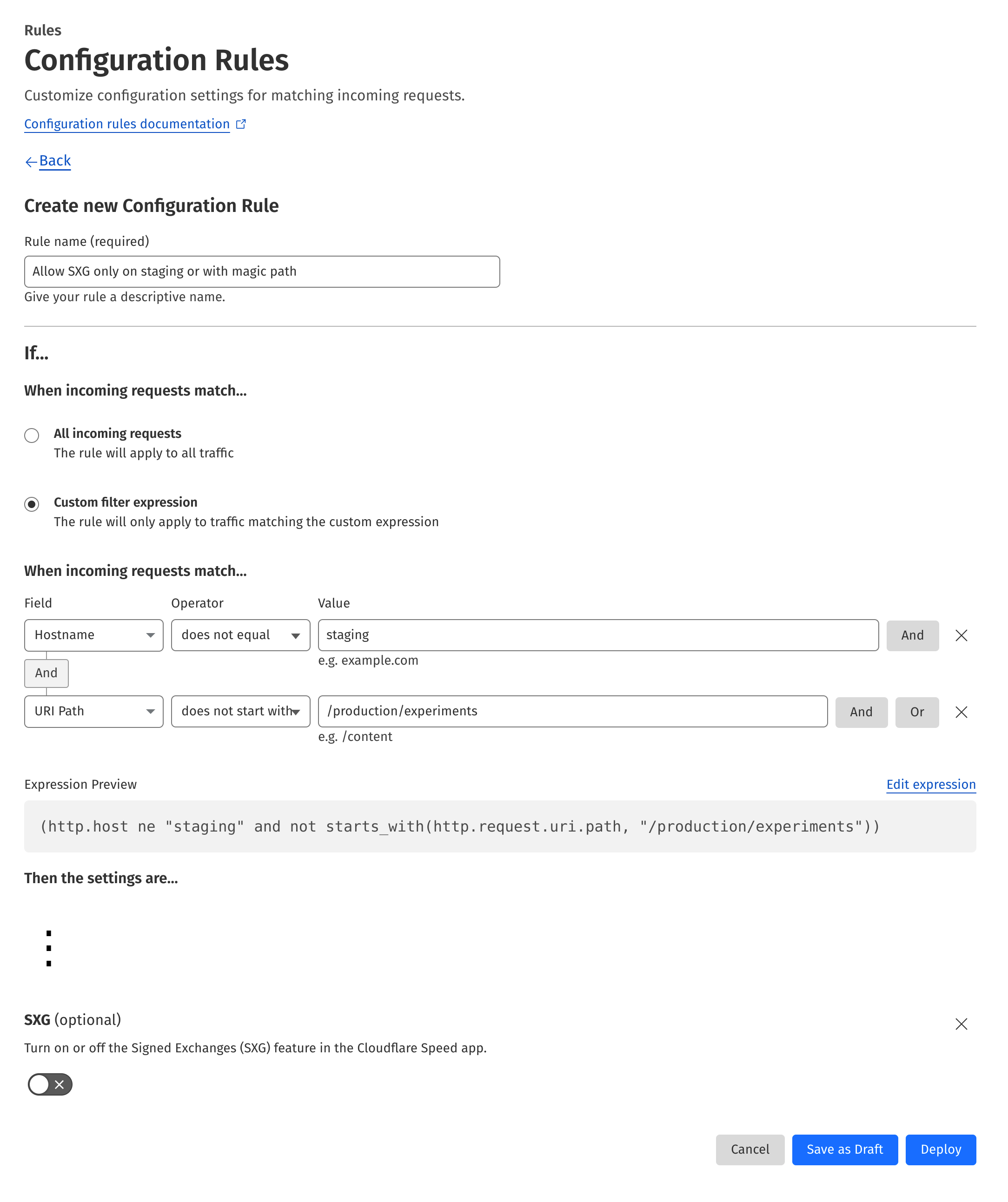The top of the page features the word "Rules" in very small type located in the upper left-hand corner. Directly below, in large, bold type, it reads "Configuration Rules." Underneath this heading, there is a description in gray type stating, "Customize configuration settings for matching incoming requests."

Following this, another line reads "Configuration Rules Documentation," with an indistinguishable emblem to its right. This text is both blue and underlined. The subsequent line has a left-pointing arrow alongside the word "Back," also in blue and underlined. 

In bold black type, the page then states "Create New Configuration Rule." Below this, it says "Rule Name (required)" followed by a rectangular input box outlined in gray with a white interior, which contains the placeholder text "ALLOW SXG ONLY ON STAGING OR WITH MAGIC PACK."

A secondary description underneath this input box advises, "Give your rule a descriptive name."

The text "If..." appears next in large, bold letters, followed by "When incoming requests match…" on the next line. There are two selection circles to choose from:
- The first circle, which is not selected, is labeled "All incoming requests" in bold letters, with the clarification "The rule will apply to all traffic" in regular black type.
- The second circle is selected and marked by a black dot in the center. It is labeled "Custom filter expression."